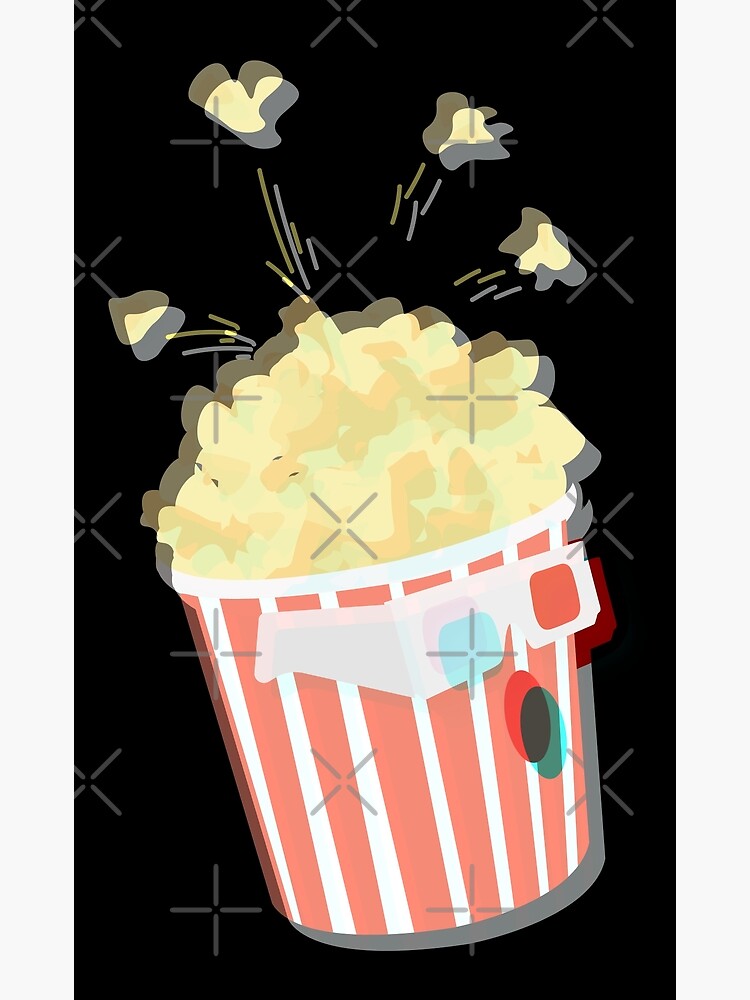The illustration features a vertical portrait of a red and white striped popcorn bucket wearing 3D glasses with red and blue lenses. Set against a black background crisscrossed with X's and plus signs, the image gives a 3D effect through a bright white afterimage slightly offset from the main elements. Golden yellow popcorn spills from the top, with four pieces dramatically popping into the air, each accented with dynamic yellow and white lines. The bucket is personified with a surprised expression, its yellow vertical oval “mouth” positioned beneath the glasses. The overall style is a playful, animated depiction reminiscent of a movie theater experience.